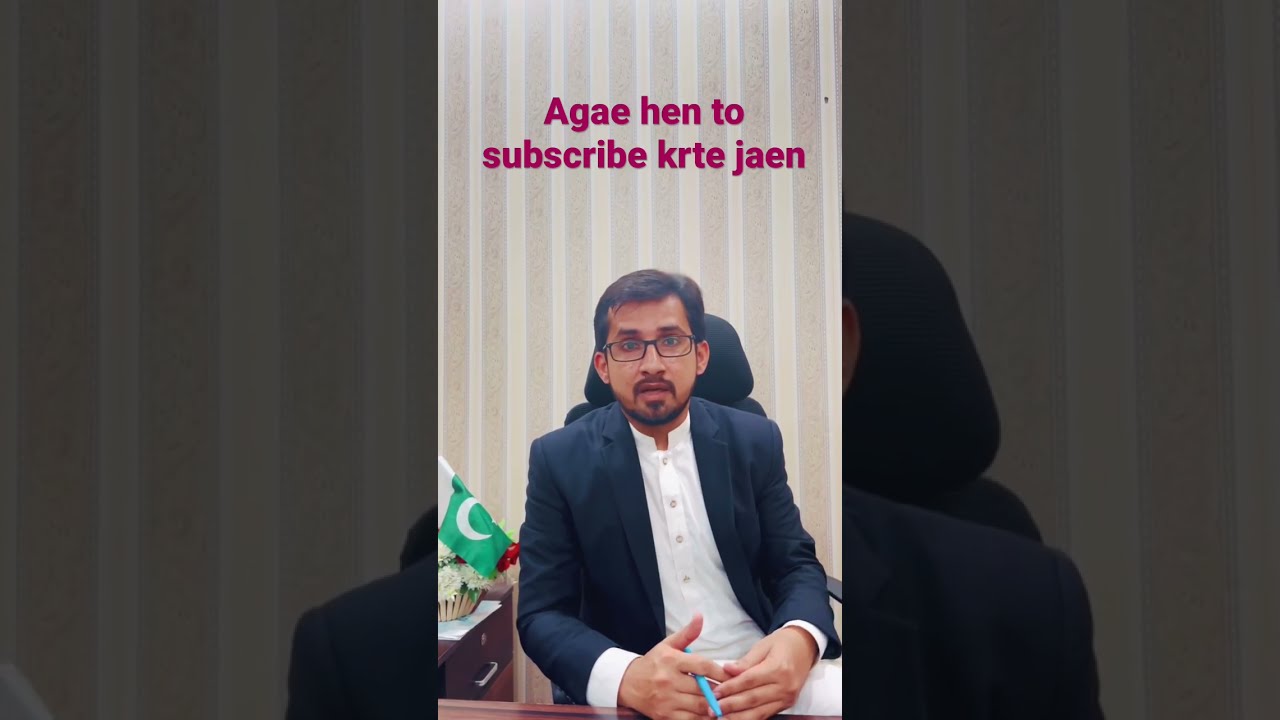The image is a screenshot of a dignified man who appears to be in his late 30s, possibly Middle Eastern or South Asian, sitting in a black cushioned computer chair. He has short brown hair, a brown goatee, and wears black-framed glasses. He is dressed in a navy blue suit jacket over a white collared shirt with buttons, holding a blue pen in his right hand. He is seated at a wooden desk with cabinets, and to his left, there is a green and white flag with a crescent moon, likely the flag of Pakistan or a similar country. The background features a wall with vertical beige and light yellow stripes. At the top of the image, magenta text reads, "If you are new to our channel, please subscribe," alongside another phrase that is less clear but seems related to a YouTube subscription prompt. The setting suggests this could be a political or religious video.